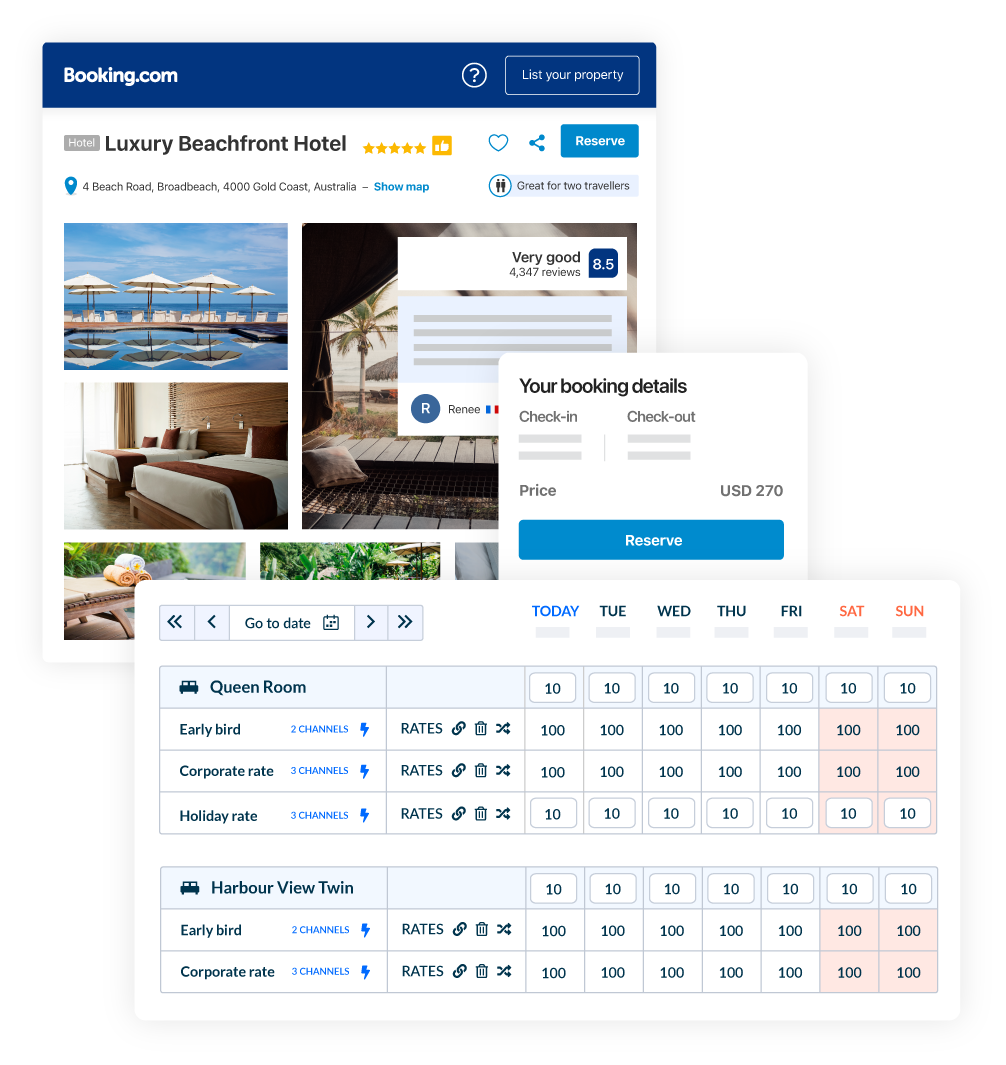Here's a detailed descriptive caption for the image:

---

The image displays the Booking.com website featuring a luxury beachfront hotel. The header contains the Booking.com logo set against a blue banner, followed by the title "Luxury Beachfront Hotel" alongside a five-star rating and a heart icon for favoriting the listing. A share button and a blue "Reserve" button follow, enabling users to book their stay. The hotel's address is listed as 4 Beach Road, Broad Beach, 4000 Gold Coast, Australia.

Below this header, several images showcase the hotel's amenities, including an outdoor pool area and a room featuring two beds. Some images are obscured by pop-ups. One prominent pop-up displays booking details such as check-in and check-out dates, pricing, and another "Reserve" button. Another pop-up beneath these details offers options to choose rooms and rates, including choices like a Queen Room or Harborview Twin Room, with various rates listed, such as Early Bird, Corporate, and Holiday rates.

---